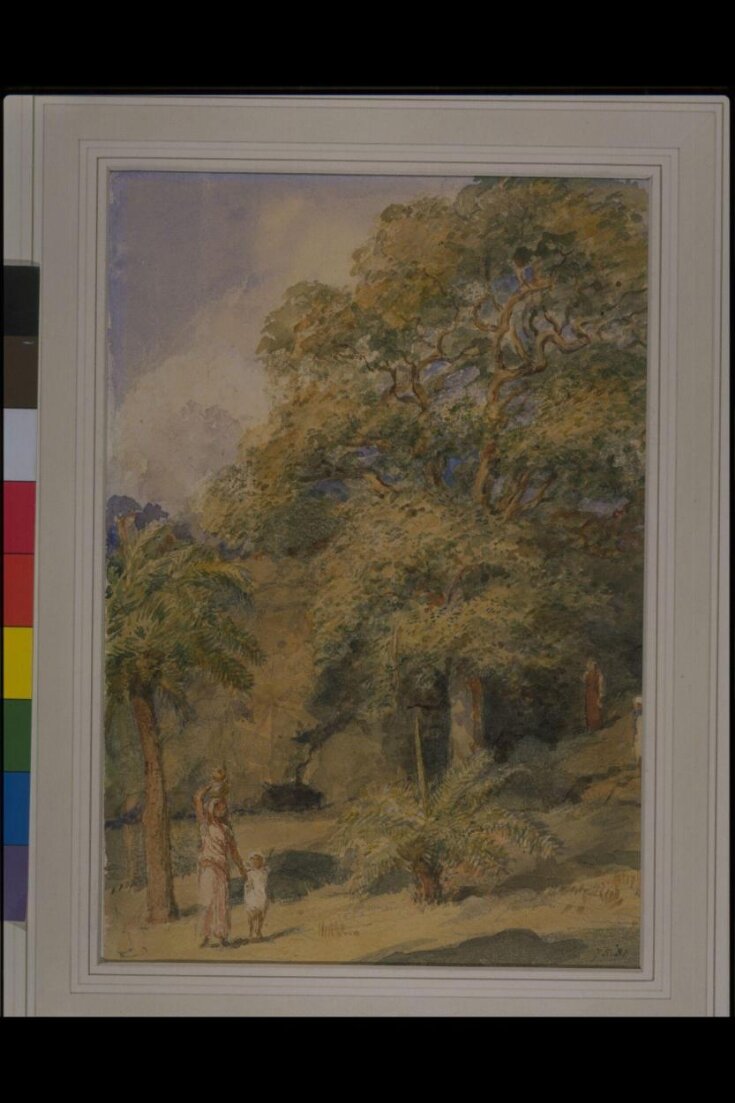This image captures a photograph of a painting set within a white wooden frame. The painting features a detailed landscape filled with various types of trees, starting with a tree resembling a palm tree in the left foreground. To the center and far right of the painting, there's a short bush, a medium-sized tree, and a very tall tree that extends to the top of the frame. In the lower left-hand corner, two figures, likely a woman and a child, stand near the palm tree. The taller figure, possibly an adult woman dressed in Middle Eastern or Biblical-style loose garments or a robe, appears to be holding objects on her head, maybe containers of water. She is holding the hand of a smaller child, who is also dressed in a white robe with a head covering. Above, a blue sky dotted with white clouds stretches across the background, with puffy clouds emerging from behind the central trees. The edges of a rainbow can be seen in the canvas's far corners, adding a touch of color to the serene scene. The ground around the figures is brownish or yellow, contrasting with the calm blue sky.